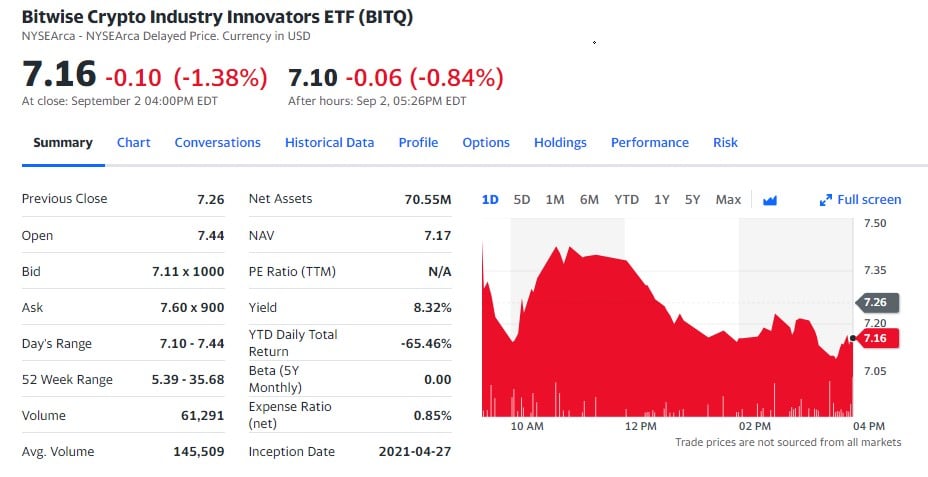This image depicts a detailed and comprehensive snapshot of a stock page for the Bitwise Crypto Industry Innovators ETF, ticker symbol BITQ, listed on the NYSE Arca exchange. The header indicates the data is in U.S. dollars (USD) and quotes are delayed.

At the center of the page, large bold numbers show the current stock price of $7.16, which has decreased by $0.10 or 1.38%, highlighted in red. Following this, the after-hours price is $7.10, down by $0.06 or 0.84%, also marked in red. Beneath these numbers, additional timestamps note "at close" values at 4:00 p.m. EDT and "after hours" values at 5:26 p.m. EDT on September 2.

A navigation bar below offers various sections, such as Summary, Chart, Conversations, Historical Data, Profile, Options, Holdings, Performance, and Risk—with "Summary" being emphasized in bold and underlined blue font.

Detailed stock information follows:
- **Previous Close:** $7.26
- **Open:** $7.44
- **Bid:** $7.11 x 1000
- **Ask:** $7.60 x 900
- **Day's Range:** $7.10 - $7.44
- **52-Week Range:** $5.39 - $68.35
- **Volume:** 61,291
- **Average Volume:** 145,509
- **Net Asset Value (NAV):** $7.17
- **Net Assets:** $70.55M
- **PE Ratio (TTM):** N/A
- **Yield:** 8.32%
- **Year-to-Date (YTD) Daily Total Return:** -65.46%
- **Beta (5Y Monthly):** 0.00
- **Expense Ratio:** 0.85%
- **Inception Date:** 2021-04-27

A graph illustrates the stock's performance throughout the trading day, with the x-axis marking 10 a.m., 12 p.m., 2 p.m., and 4 p.m. The y-axis, positioned on the right, spans values from $7.50 down to $7.05, featuring increments like $7.35, $7.26, $7.16 (highlighted in red), and $7.05. Timely markers labeled 1D, 5D, 1M, 6M, YTD, 1Y, 5Y, and MAX give options to view performance over different periods.

The line graph starts high, fluctuates, and then trends downward, depicted in red, reflecting the stock's intraday volatility.